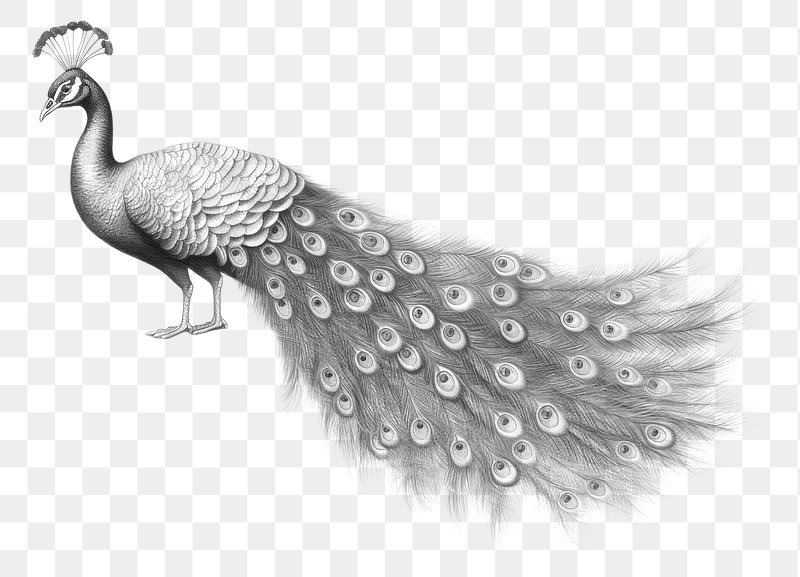The square, black-and-white digital sketch captures a male peacock in profile, facing left. Its head, adorned with a small fan of crown feathers, stands out clearly. The bird is poised with its slightly curved neck and body leading to its distinctive tail feathers, which lie flat behind it, rather than being fanned out. These tail feathers feature the characteristic "eyeball" patterns but remain devoid of any color. The background consists of a simple, pale checkerboard pattern composed of alternating light gray and white squares. The entire composition is rendered in grayscale, with no additional text, color, or artist's signature, focusing purely on the peacock and its understated elegance against the muted backdrop.